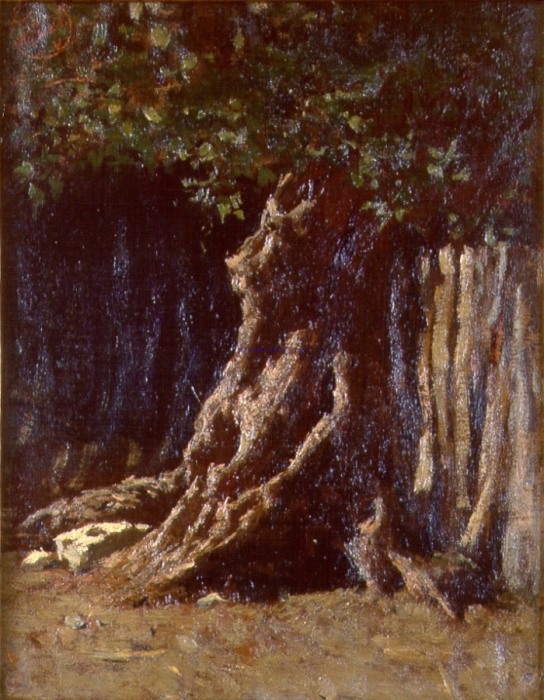This detailed artwork vividly captures an impressionist landscape featuring a dominant, aged tree at its center. The massive tree trunk, characterized by numerous gnarls, knots, and roots, spreads robustly across the brown, slightly varied earthy ground. The trunk is painted in shades of brown, yellow, and black, and it significantly broadens at the base before tapering towards the upper leafy section. The canopy is lush with a variety of leaves, showcasing a palette of green, with hints of orange, red, and brown, contributing to a vibrant, natural scene. To the right of the main tree, another thick trunk stands almost as a supporting character in this forested scenery, while patterns on the left suggest additional darker tree trunks or textured shadows. The background hints at an abstract, forest-like setting, potentially blending in elements of rock or granite, giving depth and context to the primary tree's grandeur. The painting’s abstract and impressionist elements create an evocative, nature-inspired scene, devoid of any human or animal life, focusing solely on the splendor of the tree and its surroundings.